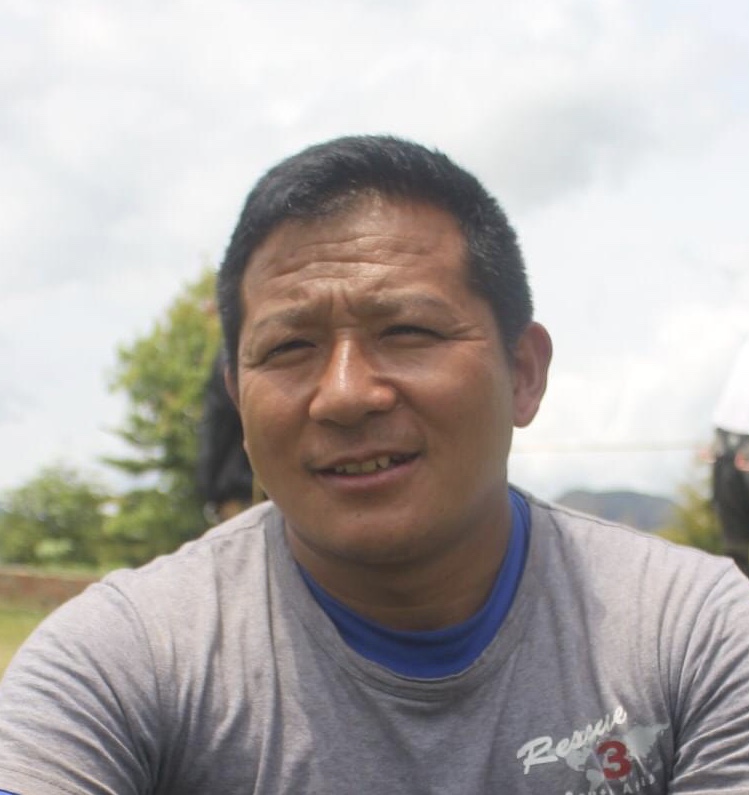The image features a man of medium skin tone with short, slightly brown-tinged black hair, estimated to be around 35 to 40 years old and possibly of Asian descent. He is outdoors, smiling gently and squinting at the camera, suggesting it may be sunny out. He is dressed in a layered outfit consisting of a blue t-shirt beneath a gray t-shirt. The gray t-shirt is distinctive, featuring an iron-on image that includes the word "Rescue," the number "3" in red, and a map of the world in white. The background is somewhat blurred but shows a green field, a few trees, and an expanse of sky that is partly cloudy with blue patches. There is a hint of other elements such as a potential billboard and indications of hills or mountains in the distance. The presence of other people is uncertain due to the blurriness, although there might be a couple of indistinct figures in the background.